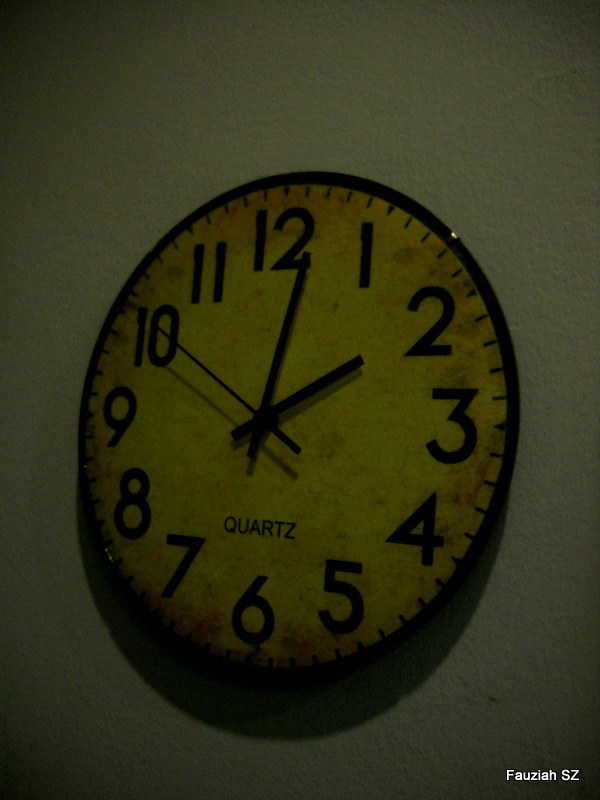This color photograph features a vintage circular wall clock against a textured wall that appears medium gray due to underexposure. In the bottom right corner, the text "FAUZIAH SZ" is displayed in a bold white font. The clock's face, originally yellow, shows signs of aging with scattered brown discoloration. Black numerals and the word "quartz" are clearly visible beneath the hands, which indicate the time is 2:01. The clock is encased in a black circular frame, adding contrast to the overall dark aesthetic of the image.